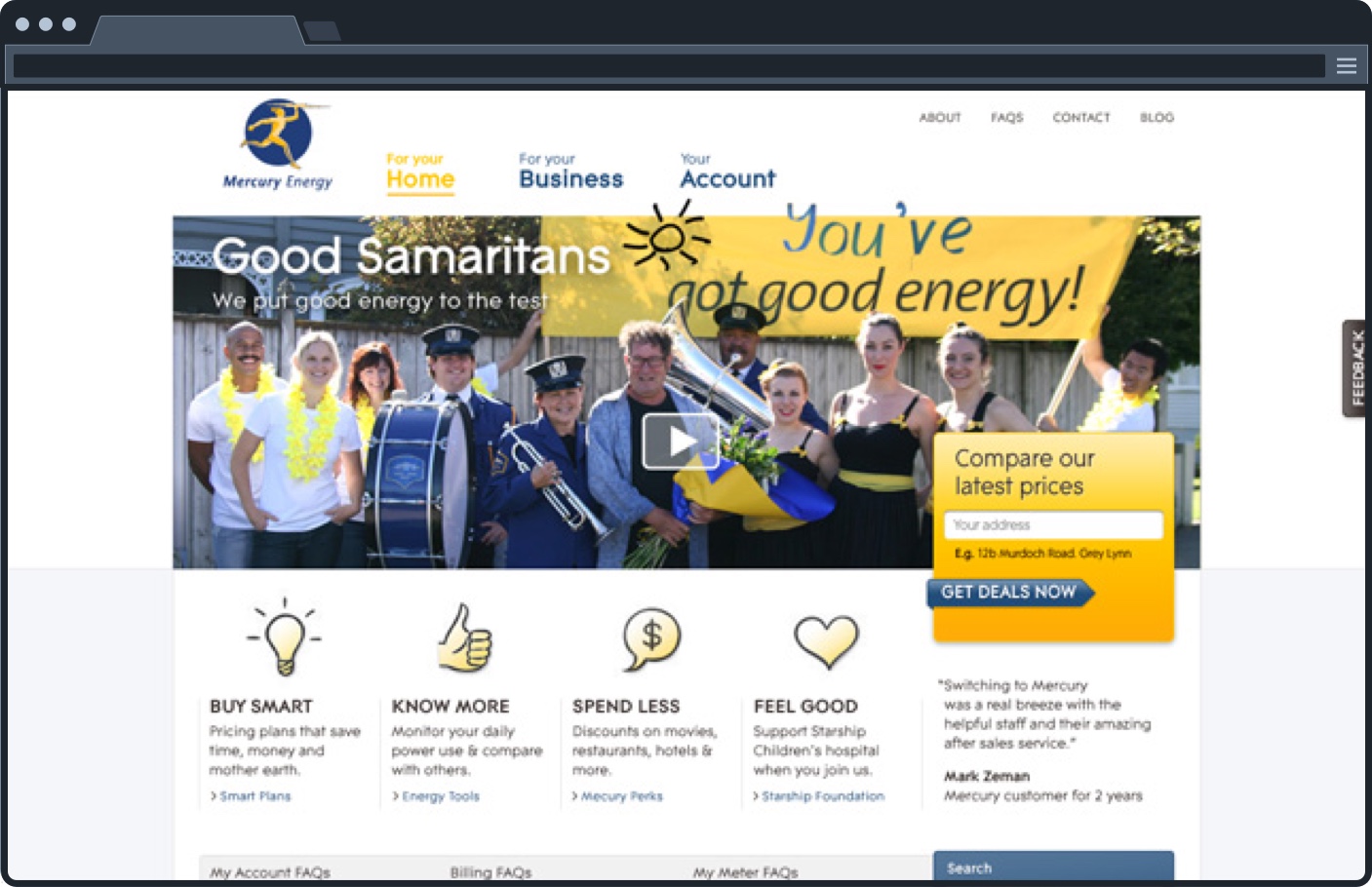The image depicts a webpage viewed on a Mac interface.

At the top, there's a black header featuring three gray buttons or letters on the left-hand side, resembling standard browser navigation elements. The address bar is completely blackened out, while towards the right-hand side, three horizontal gray lines are visible.

Below, a vibrant banner dominates the screen. On the left side of the banner, an orange figure that appears to be running is surrounded by a blue background. Adjacent to this figure, the text reads "Mercury Energy" in white. Below it, additional text, "For your home" in yellow, and "For your business" in blue, is prominently displayed. Further along, the banner mentions "Your account" in smaller text.

In the upper right corner of the page, categories like "About," "FAQs," "Content," and "Blog" are listed in a smaller font.

The central portion of the image captures a group of people standing around with band equipment. The individuals are dressed in white, blue, and black, suggesting a casual, yet coordinated appearance. A yellow banner is displayed behind them, and a digitally added sun with the phrase "You Got Good Energy" appears, albeit with a noticeable typo presenting as "You've not good energy."

Beneath this visual, a yellow square contains the text "Compare our latest prices" in black. An adjacent address bar, where users can presumably type information, is labeled with "Great deals now" and slogans such as "Smart No More," "Spend Less," and "Feel Good."

Overall, the image seems to revolve around promoting an energy service, emphasizing its applicability to both home and business, and encouraging engagement with various features and deals.